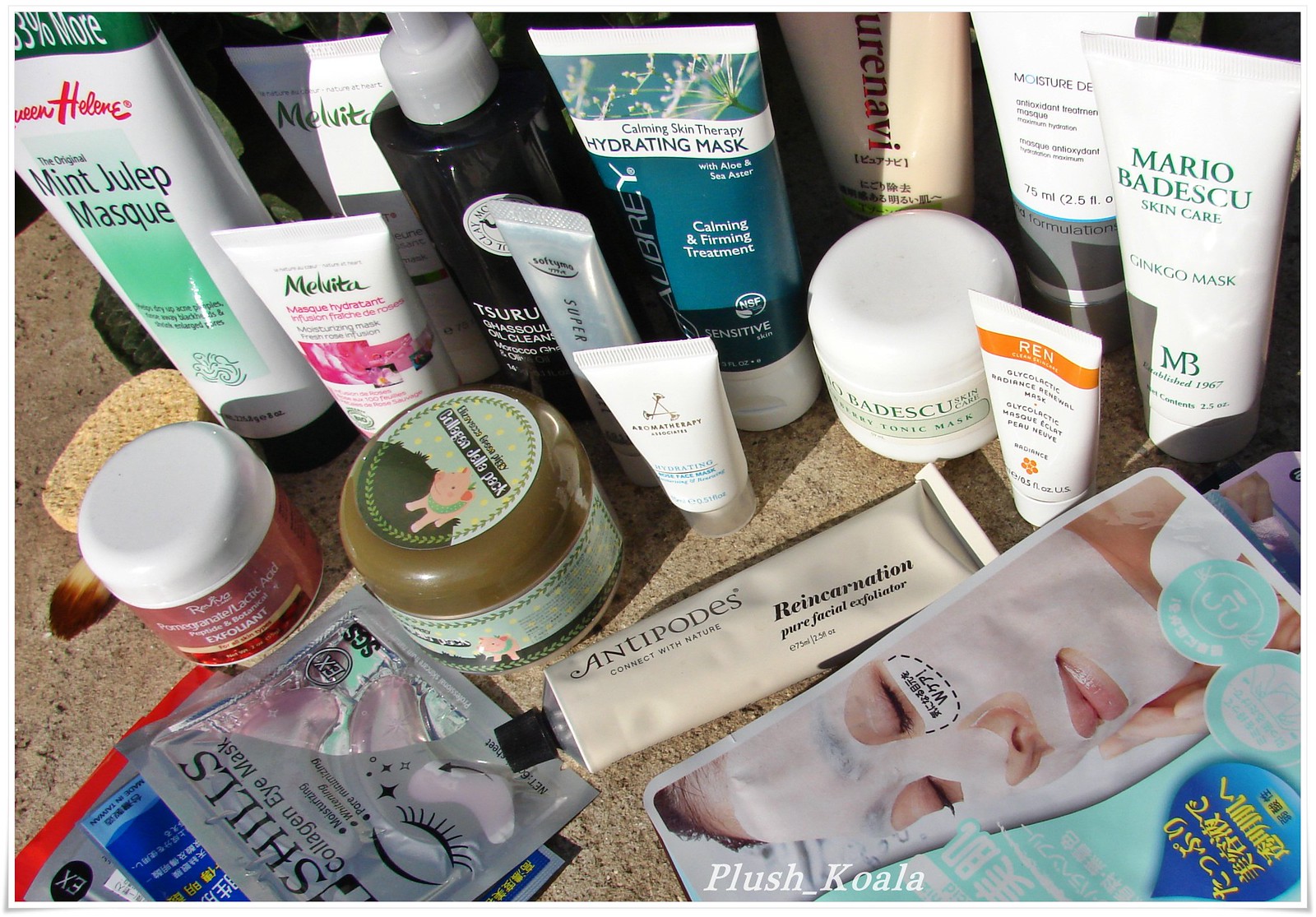A meticulously arranged collection of health and wellness skincare products sits atop a pristine surface, showcasing a variety of items. On the left, a couple of tubes catch the eye, including the "Mint Julep Masque" by Helene, characterized by its distinctive white and green packaging. Adjacent to it are several products from Melvita, presented in elegant white tubes adorned with delicate floral designs, although their specific purposes remain indistinguishable. Smaller items punctuate the setup, among them a series of exfoliants and various sachets in shades of gray and blue.

Prominently displayed is a face mask featuring a woman's serene visage, adding a touch of personalization to the assortment. The “Antipodes Reincarnation” facial cream stands out, promising rejuvenation. Not far from it, a hydrating mask joins the ensemble, further emphasizing the theme of skin nourishment. Notably, two products from Mario Badescu are visible: the larger Ginkgo Mask and a smaller item from the same brand.

This curated selection of facial products highlights a comprehensive skincare regimen aimed at maintaining a healthy and clear complexion. The variety underscores a commitment to thorough skincare, with options for hydration, exfoliation, and rejuvenation.